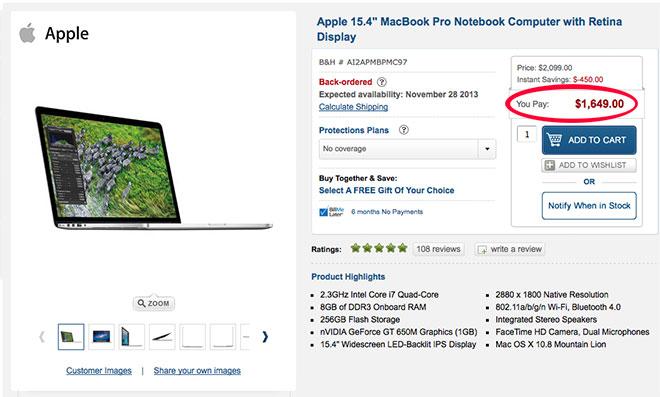The image depicts an Apple Store webpage featuring a product listing for the Apple MacBook Pro notebook. The webpage background is a light gray color. On the left side, there is a prominent white square section displaying the iconic Apple logo and the word "Apple" in the top-left corner. Below, there is an image of the Apple MacBook Pro notebook, accompanied by several smaller thumbnail images underneath that offer different viewing angles when clicked.

On the right side, at the top of the section, the product description reads "Apple 15.4-inch MacBook Pro notebook computer with Retina display." It is noted that the item is back-ordered, with availability expected on November 28th, 2013. A button labeled "Calculate Shipping" is available, along with information on protection plans and a financing option that allows for six months of payments with no interest.

The original price of the MacBook Pro is listed as $2,099, with an impressive instant savings of $450, bringing the price down to $1,649. There are buttons for "Add to Cart" or "Notify When In Stock." Beneath this, the product has received an average rating of five stars based on 108 reviews. At the bottom of the section, there are product highlights summarizing the key features of the MacBook Pro.